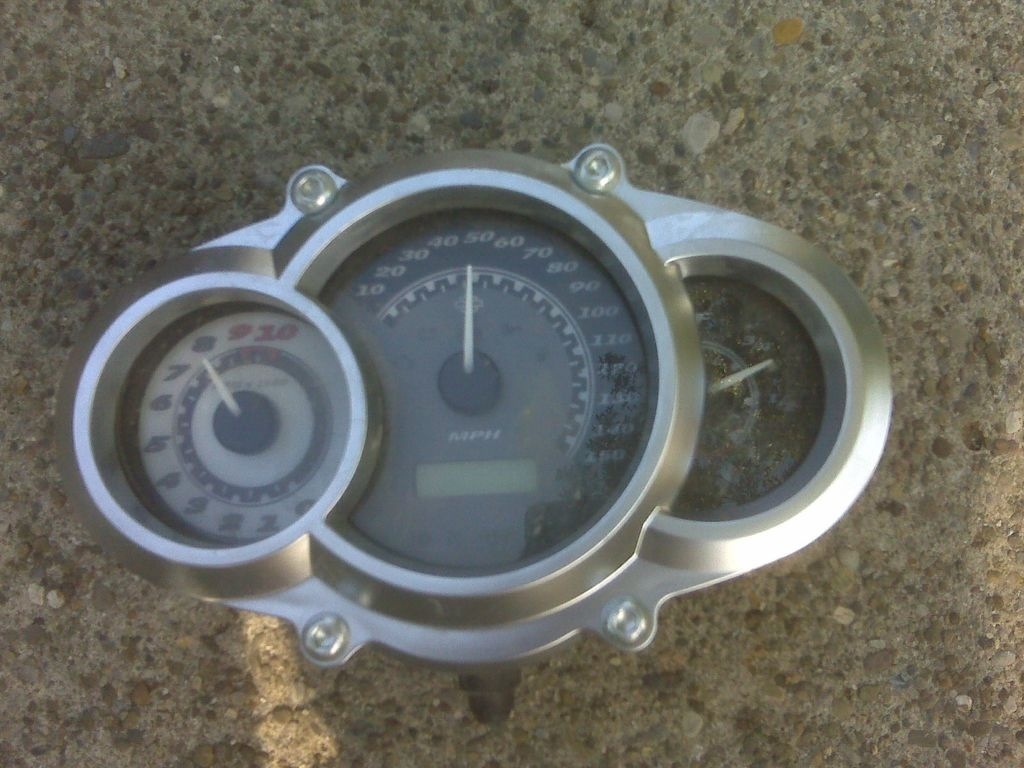The photograph showcases a speedometer assembly likely extracted from a motorcycle, placed on a surface that appears to be either a granite countertop or a textured cement ground made up of small rocks, suggesting a rugged or industrial setting. The speedometer device consists of three circular dials arranged in a slightly overlapping pattern:

1. The left dial features a scale ranging from 0 to 10, marked from the bottom left clockwise, with sections 0 through 8 in black and 9 and 10 in red, indicating it might measure RPMs with the red section representing the higher, potentially dangerous range.

2. The central dial is the largest and displays speed in MPH, with a scale running from 10 to 150. It also incorporates a small green digital screen below the speed marks, likely showing the odometer reading or additional information.

3. The right dial, smaller and partly obscured by dirt, seems to be an oil level indicator.

All three dials are encased in a weathered and dusty exterior, suggesting they were actively used before being disassembled. The varying sizes and specific functions of the dials hint at a well-engineered instrument cluster designed for a motorcycle, offering crucial information at a glance to the rider.